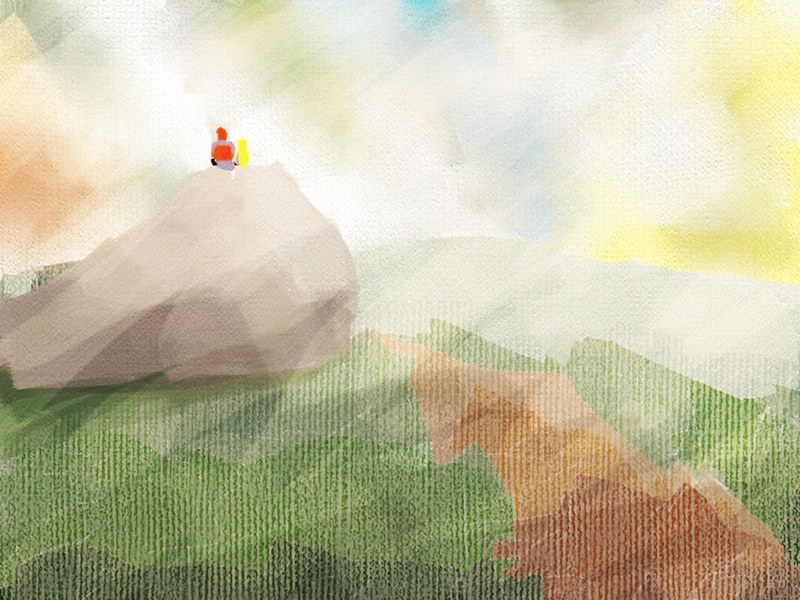This image appears to be a detailed, colored artwork, possibly a painting or illustration, characterized by its distinctive texture suggesting it might be on canvas. The scene depicts a bright green grassy plain or low hills, using a range of green shades from light to dark. Dominating the foreground is a large, light gray boulder, approximately 15 feet tall, providing a perch for two small figures whose backs are turned to the viewer.

The first figure has orange hair and appears to be holding a small, light gray sword, while the second, smaller figure is likely female or a smaller friend with blonde hair, dressed in red and white. Above them, the sky is rendered in unexpected streaks of color: browns, bright whites, greens, blues, yellows, and a touch of blue, creating an unusual and striking backdrop. The image conveys a sense of peaceful observation, with detailed brush strokes and a gritty texture enhancing its artistic depth.